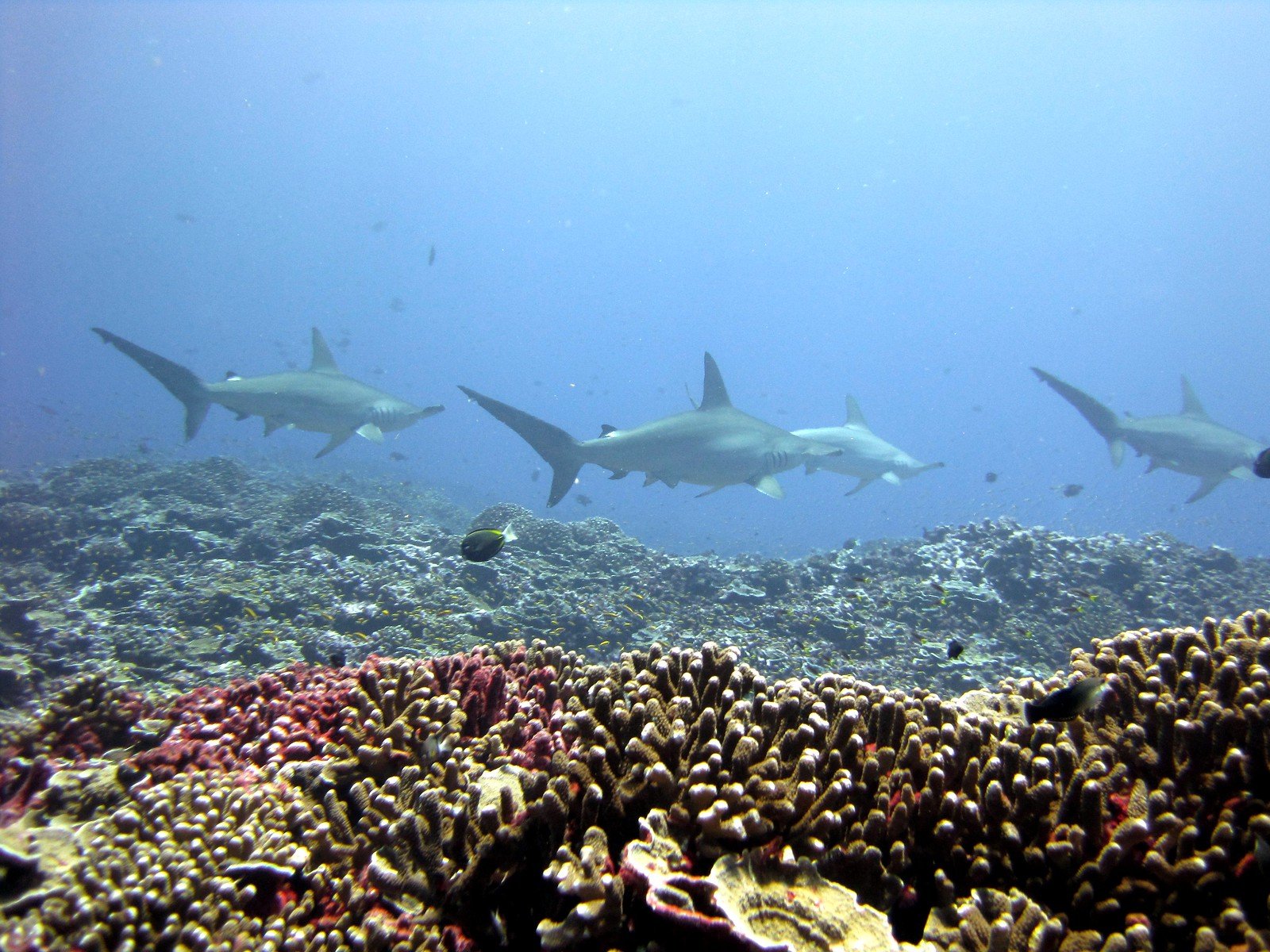The image captures an underwater scene at the bottom of the ocean, showcasing a coral reef adorned with muted dark brown and purple hues mingled with beige, red, and blue patterns. In the mid-ground, four sharks, possibly resembling hammerhead sharks, swim from left to right. The sharks vary slightly in size due to their depth in the scene, with two appearing larger and two smaller, set against the darker coral below them. These dark-colored sharks feature noticeable long dorsal fins and faint shadows of their hammerhead shapes. Additional smaller fish, including a yellow flounder-like fish, swim alongside the sharks. The upper half of the image reveals a clear blue expanse of water, slightly murky, hinting at the light from above. Rocks and other marine structures are scattered in the background, contributing to the vibrant and intricate underwater landscape.